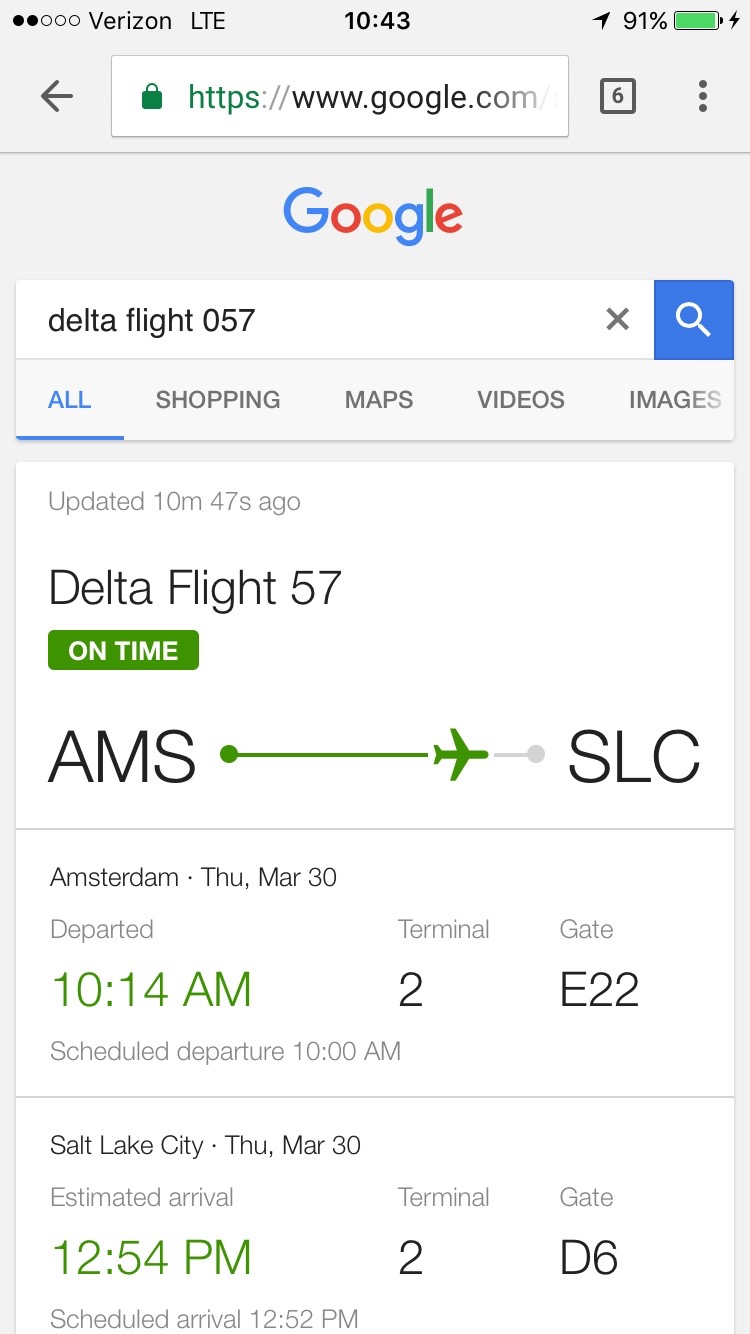The image is a phone screenshot of a Google search. At the very top right, there is a black lightning bolt icon, and to its left, a green battery icon that indicates the battery is 91% charged. There's also a location icon to the left of the battery, resembling an arrow pointing to the top right. In the top center, the current time displayed is 10:43.

Below this, the URL reads "https://www.google.com". Underneath the URL, the Google logo is displayed in its characteristic colors: blue, red, yellow, blue, green, and red. Centered below the logo is the search bar, containing the text "Delta Flight 057".

The interface then shows several category options with "All" highlighted in blue and underlined. To the right are categories labeled "Shopping," "Maps," "Videos," and "Images".

Below this section, flight details are visible. It notes the information was updated 10 minutes and 47 seconds ago and concerns Delta Flight 57. A small box indicates the flight status as "On Time". Further down, "AMS" and "SLC" are displayed with a green line between them, and an airplane icon points from Amsterdam (AMS) to Salt Lake City (SLC).